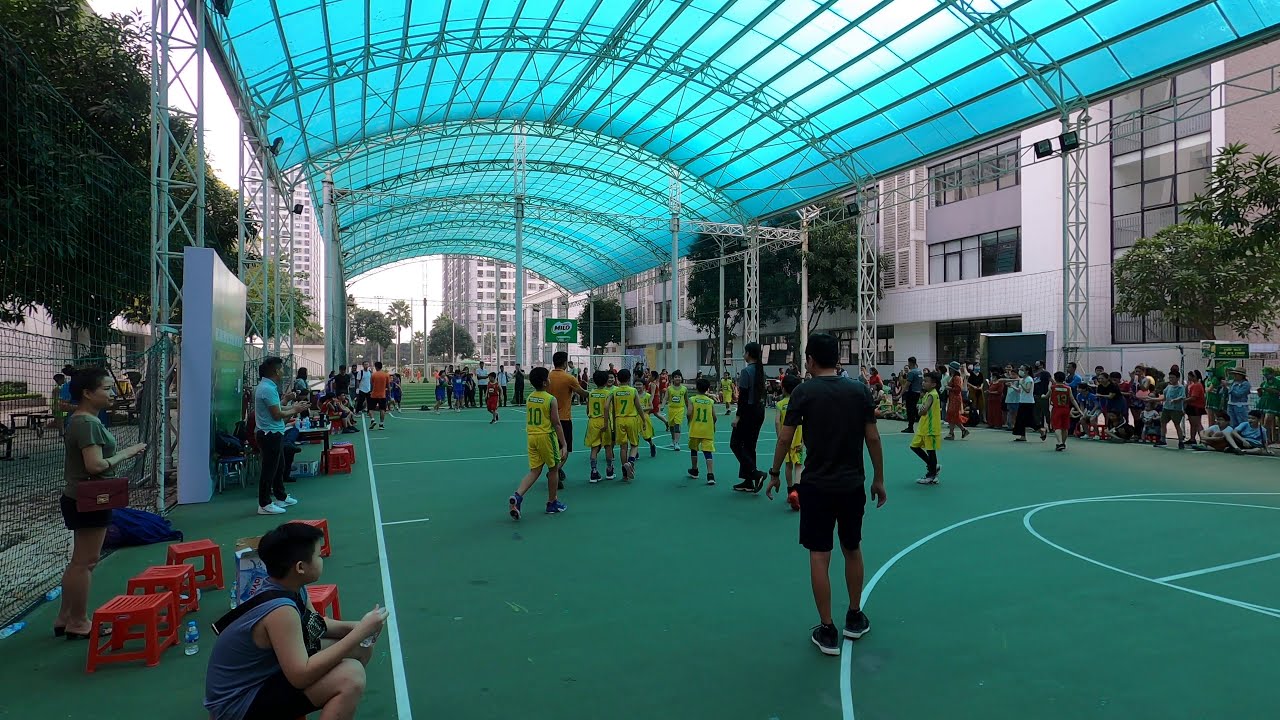The image portrays a lively children’s Milo basketball competition set in an outdoor yet fully shaded court. The court, painted green with white lines, is situated under a blue awning supported by wire frames, creating a well-lit but shaded environment. Central to the image are children gathered in yellow sleeveless jerseys with green numbers, indicative of a team, while others sport red jerseys. A noticeable man in black attire and black sneakers with white soles stands out among the group. Toward the left, a boy in a blue sleeveless jersey is seated, accompanied by a lady adorned in a green t-shirt, black shorts, and carrying a red handbag. Another prominent figure is a lady in a blue t-shirt, long hair, black trousers, and black sneakers positioned centrally. The area is encircled by tall, white buildings adding to the urban ambiance, with Milo signage subtly visible in the background. Additional details include small red stools characteristic of those found in Vietnam, hinting at the location’s cultural setting.